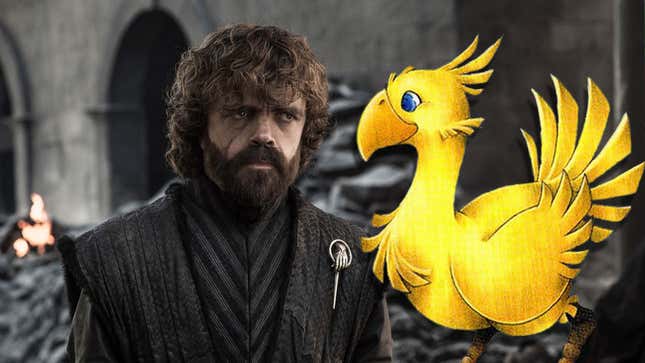The image is a still from Game of Thrones featuring Peter Dinklage as Tyrion Lannister. Tyrion, with his longish brown curly hair and beard, is dressed in a grey striped shirt with a thick grey vest over it, and has a pin on the front of his garment. He stands in front of blurred stone buildings with arched doorways, with a small fire visible on the left side near the bottom. Tyrion has a sad, contemplative expression as he looks off to the right. Superimposed discordantly on the right side of the photograph is a bright yellow cartoon duck with blue eyes and an orangish beak. The duck appears cheerful and is looking directly at Tyrion, creating a surreal and contrasting image.